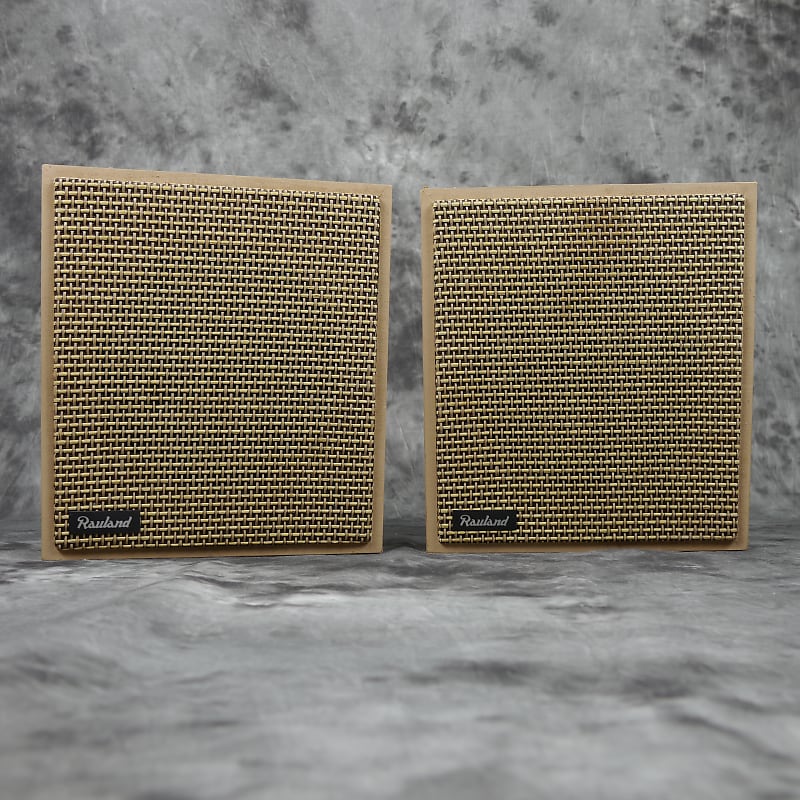In this realistic picture, two vintage-style speakers are prominently displayed against a backdrop of gray and white patterned fabric that mimics a marble surface. Each speaker is a light tan square with a raised, woven mesh design covering most of the front. This mesh is a mixture of tans and lighter browns, creating an intricate, textured appearance. Both speakers feature a small, black nameplate in the lower left corner, bearing the name "Rauland" in cursive lettering. The backdrop and floor both carry the same gray and white marble-like pattern, with the backdrop having more dark gray or black splotches compared to the surface the speakers are sitting on.